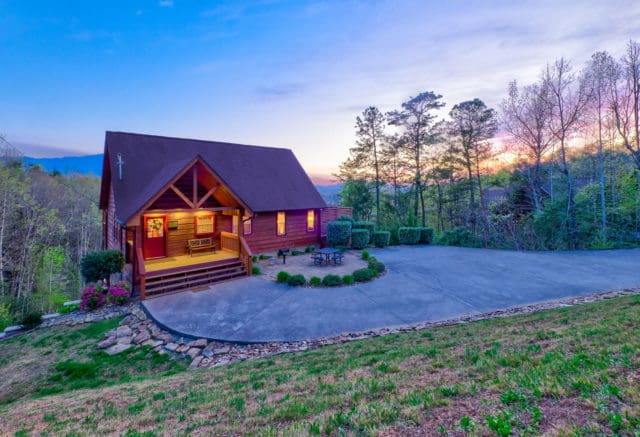The photograph captures a secluded log cabin, surrounded by a wooded area, during twilight with an unusual coloring. The cabin features a dark, pointy roof, possibly black, and a red door accessed by four brown wooden steps with railings, leading up to a small front porch illuminated by a light. The porch also has a brown wooden bench. The warm glow from the windows and porch light contrasts with the dimming sky, which transitions from blue to a pinkish hue with feathery white clouds. The front yard of the cabin includes an area that appears to be macadam, tinted blue by the sunset. Surrounding this space are stones in shades of white, black, and tan, alongside finely cut bushes and some greenery. The scene also depicts a picnic area with a grilling pit and a black or green table with attached seats. The lush environment extends to a grassy hill and clusters of trees, some vibrant green and others with reddish tones, set against mountain ranges that appear blue in the background. The overall setting conveys a serene and picturesque retreat amid nature.